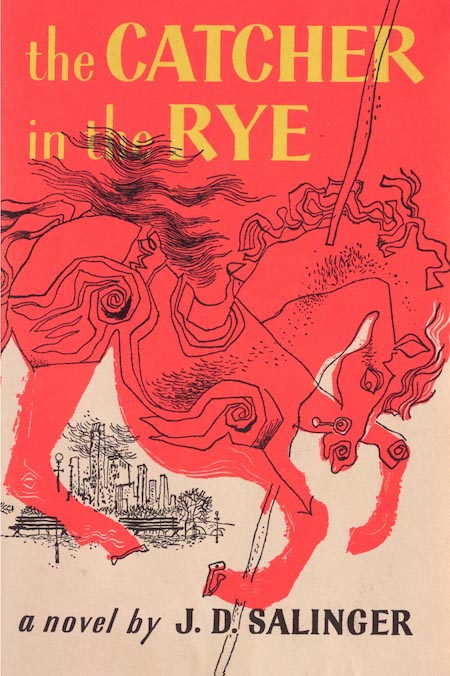The cover of the book "The Catcher in the Rye" features a striking design blending abstract artistry with bold typography. Dominating the top portion is the title, "The Catcher in the Rye," rendered in eye-catching yellow text, utilizing a mix of uppercase and lowercase letters. This sits against a dynamic red backdrop, which transitions into a calm beige tone toward the bottom of the cover. The centerpiece of the design is an abstract hand-drawn illustration—a pen line drawing of a carousel horse. This horse is intentionally misproportioned and features a series of swirls and intricate lines, blending seamlessly with the lower cream-colored portion of the cover where additional elements of a cityscape, possibly resembling Central Park, are sketched in a similar style. At the bottom left corner, the cover is signed off with the words "A Novel by J.D. Salinger," confirming the author's identity. The overall effect of the cover is both intriguing and visually appealing, capturing attention with its bold colors and distinctive art.